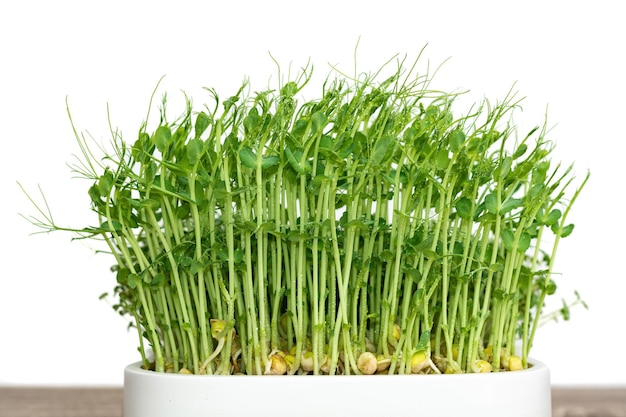This highly detailed close-up photograph features a dense cluster of vibrant green microgreens or sprouts, most likely an herb due to their delicate structure. The sprouts, packed tightly together, are growing in a circular white dish, only the uppermost half-inch of which is visible. The background behind the sprouts is predominantly white, with slight brownish blurs at the periphery, possibly indicating a wooden table surface the dish rests upon.

Each sprout stands tall, reaching upwards with long, light green stalks that support a few small, dark green leaves near their midpoints, with more foliage and fine, wispy extensions crowning the tops. These textures create a thick, almost impenetrable forest-like canopy, though the lower parts of the stalks provide glimpses of a white background.

At the base of the stalks, small, yellowish-white, mushroom-like seed pods are visible, from which the microgreens sprout. This combination of vibrant green stems, delicate leaves, and the earthy-toned seed pods offers a rich, textural contrast within the small, contained garden.